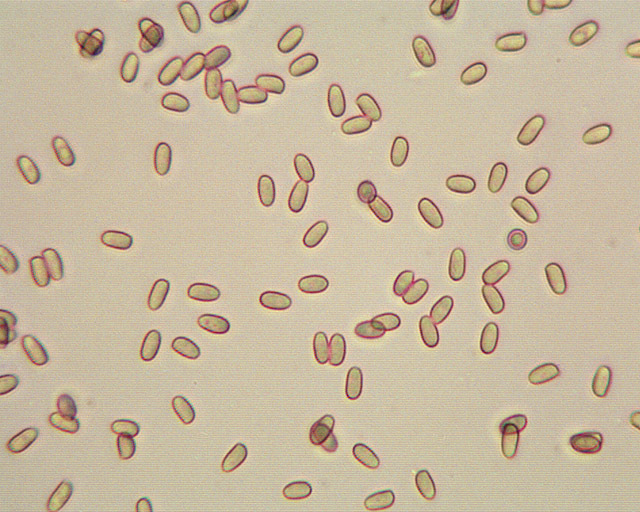This highly magnified image depicts numerous small, oval-shaped objects scattered across a beige background. Resembling a mix of beans or Tic Tacs, each of these ovals is surrounded by a distinctive red or sometimes fluorescent purple outline, with greenish-yellow interiors. The objects appear randomly distributed, without any discernible pattern or order, and some seem embedded into the background. No additional text, watermarks, or dates provide further context, lending the image an abstract, experimental feel, reminiscent of materials seen in a science classroom or an educational video. The detailed microscopic nature of the image suggests these oval forms could be cells, contributing to the image's scientific aura.